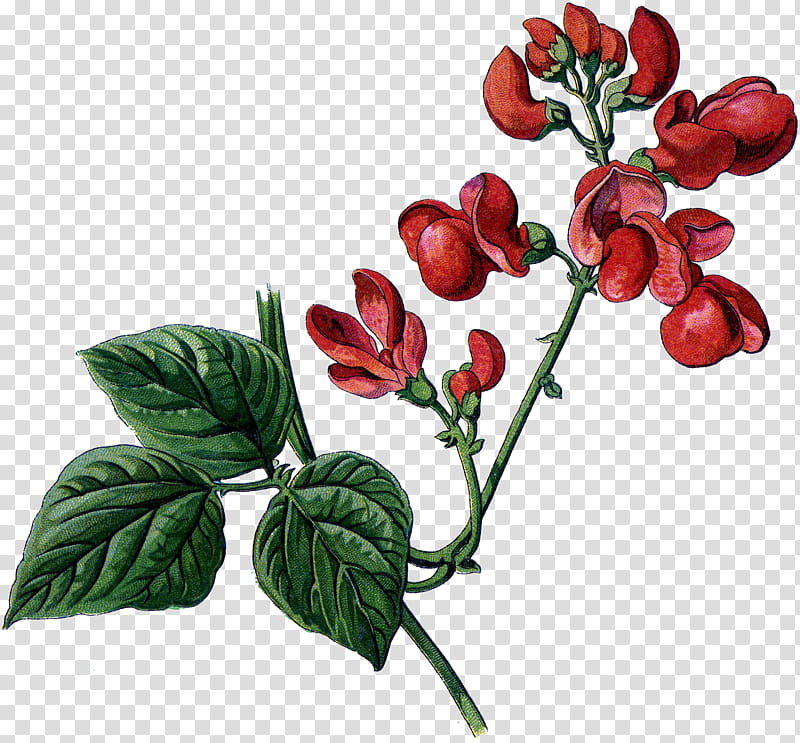The image is a digitally generated drawing of a plant set against a white and gray checkerboard background, resembling a chessboard with small checks. The plant features green, large leaves and multiple green stems. From these stems sprout vibrant red flowers, some of which are in full bloom, while others appear as either budding flowers or chili peppers. The meticulous detailing of the textures on the leaves and petals is evident, suggesting a digitally printed design. The plant's primary thick green stem curves gracefully and connects to a larger plant that fades off towards the bottom, adding a dynamic visual flow to the composition.